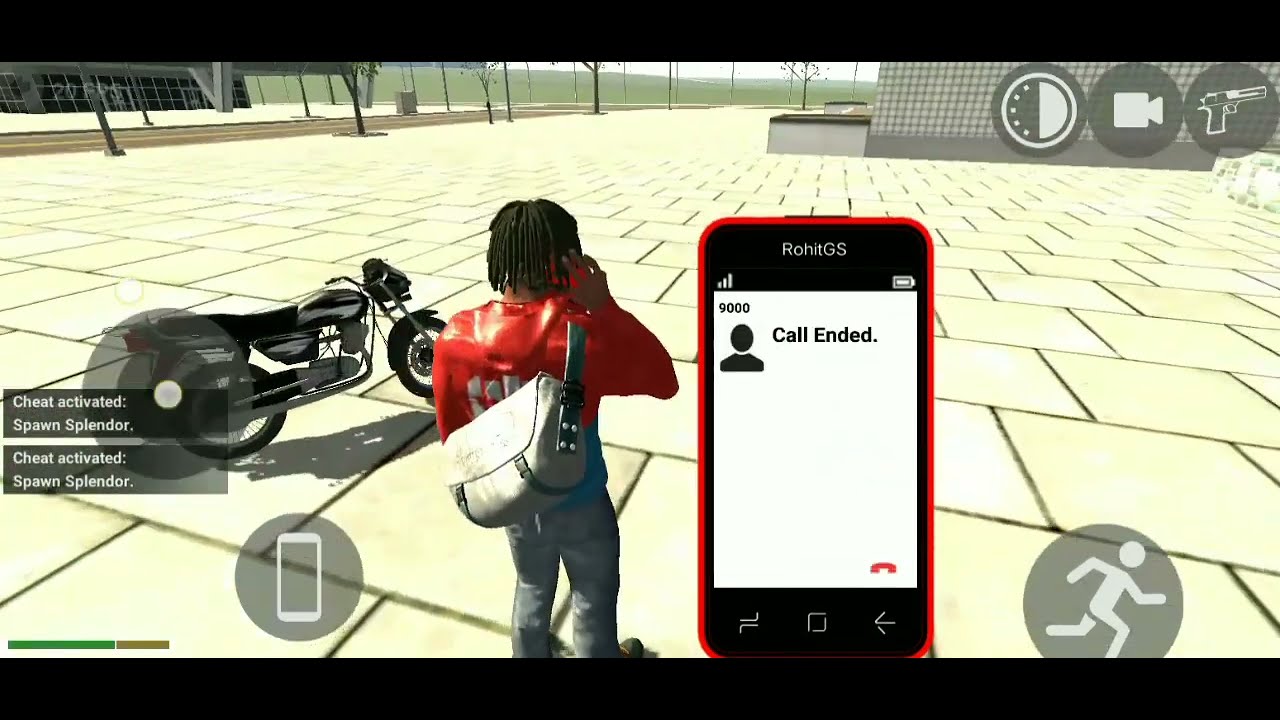This is a horizontally aligned rectangular image, seemingly a screenshot from a mobile video game displayed in landscape mode with thick black borders at the top and bottom. The setting appears to be a large, open sidewalk area paved with square beige tiles, reminiscent of a college campus. The focal point of the image is a black male character, viewed from behind, who is wearing a red top or jacket, gray pants or jeans, and has a large knapsack bag slung over his back. His hair is worn in short braids or dreads that reach down his neck. To his right, there is an image of a cell phone with a white screen and a red border that reads "Call Ended," similar to an early iPhone interface. To his left, a motorcycle is parked. There are two duplicate boxes floating nearby, each with the text “Cheat activated, spawn Splendor.” In the background, trees and some grass are visible.

The screen also features typical mobile game icons. On the left side, there is a joystick for movement, while at the bottom right, there is a sprint button depicting a running figure. The top right corner hosts additional icons, including what looks like a sun and a camera, the latter resembling a video chat option, and a pistol icon, indicating weapon selection. These icons are placed within gray-like surroundings.